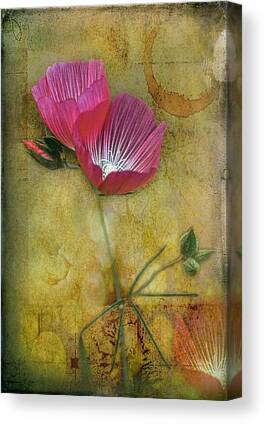This photograph captures an abstract, oil-painted canvas that exudes a rich artistic essence. Dominated by a weathered, yellowish-brown background featuring subtle water spots and orange hues, the canvas creates a compelling juxtaposition for the vibrant subject it frames. Central to the composition are two prominently featured pink or fuchsia poppy-like flowers, each boasting striking white centers and detailed long-stripe patterns on the petals. The flowers are set off by a robust, green stem that branches out to include smaller buds and closed blossoms, adding to the depth of the piece. The painting’s texture stands out, appearing almost as a high-quality print stretched over a wood frame, approximately two inches thick, making it ready for display in spaces like a hotel or kitchen. The overall effect draws the viewer's eye to the colorful, centrally-placed flowers, making them pop against the muted, yet artfully weathered backdrop.